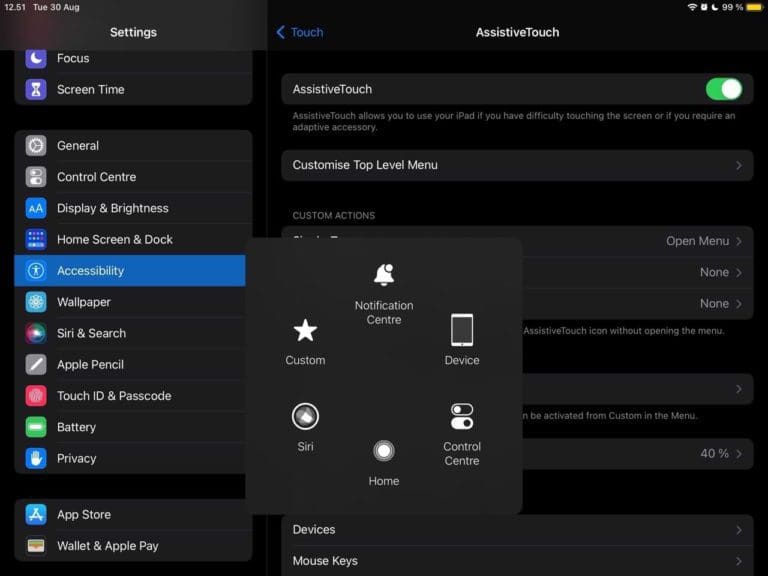This screenshot, taken on an Apple iPad in horizontal mode on Tuesday, August 30th at 12:51 PM, depicts the device's Settings application. The time and date are prominently displayed in the top left corner, while the top right corner indicates the device is connected to Wi-Fi, has a 99% battery level, and is in Low Power Mode.

The screenshot focuses on the Accessibility section of the settings, specifically highlighting the activation of the AssistiveTouch feature. Once enabled, a large square interface appears in the center of the screen, organized in a circular formation with various icons and labels. At the top of this interface is the "Notification Center" icon, followed by "Custom" to the right, "Siri" below, "Home" to the right of Siri, "Control Center" to the right of Home, and "Device" above Control Center.

On the left side of the screenshot, a vertical list displays other available settings options the user can navigate through. These options include Focus, Screen Time, General, Control Center, Display & Brightness, Home Screen & Dock, Accessibility, Wallpaper, Siri & Search, Apple Pencil, Touch ID & Passcode, Battery, Privacy, App Store, and Wallet & Apple Pay.